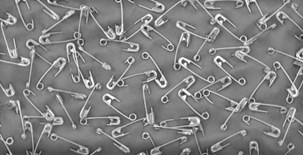The image presents a small, narrow landscape photograph of numerous safety pins scattered over a charcoal gray fabric background. Each silver safety pin casts distinct shadows onto the dark fabric, emphasizing the contrast and adding a sense of depth to the arrangement. The pins are in various states of openness, pointing in all different directions, and many are overlapping or touching at different angles. The background appears slightly wrinkled, further adding texture and realism to the composition, which appears almost as a piece of abstract art. All safety pins are of the same size, clean, and shiny, contributing to the overall cohesion and detail of the image.